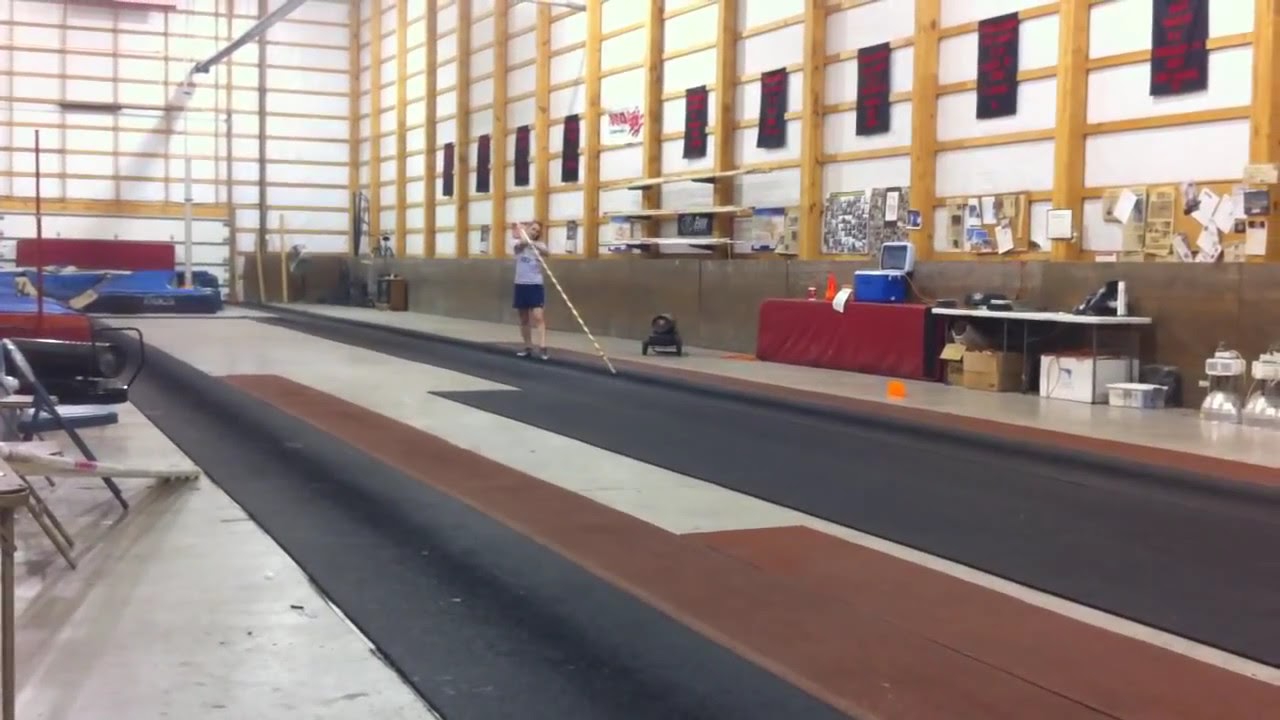In this detailed photograph, a girl stands poised in an indoor arena, ready to execute a pole vault. She grips a long, yellow pole with one arm while standing on a narrow, dark runway. She is dressed in a gray short-sleeve t-shirt, navy blue shorts, and sneakers. The long, black runoff strip leads toward cushioned blue mats where she will land after her vault.

The arena itself is spacious and framed with a distinctive grid-style wooden structure, giving it a warehouse-like appearance. On the right, there's a red table with a blue cooler, surrounded by various gym equipment including a fan and boards with notices. On the left, additional mats are visible alongside folding chairs and more gym equipment. Hanging from the vertically and horizontally lined wooden walls are black banners adorned with red text, enhancing the athletic atmosphere of the space. The entire scene is an encapsulation of a dedicated athlete preparing amidst a backdrop of organized yet bustling gymnasium elements.